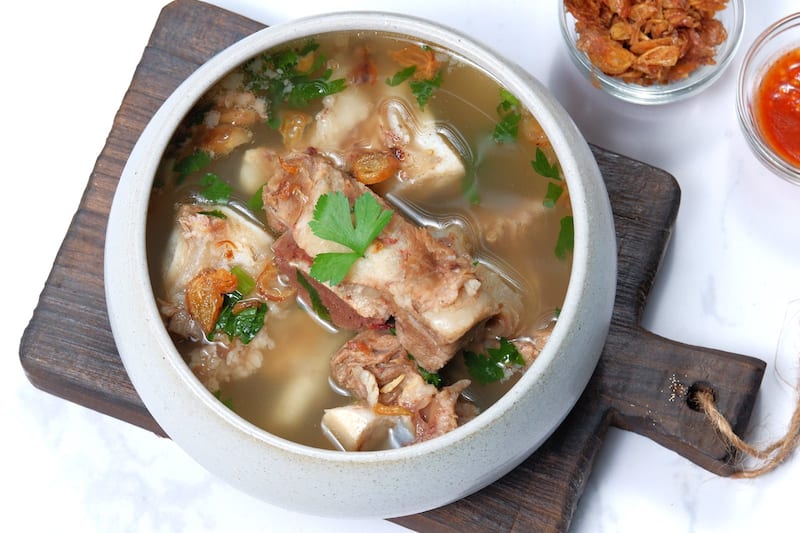The image depicts a close-up of a white ceramic bowl filled with light brown broth that resembles pho, showcasing a mixture of meat—likely pork or beef—and garnished with fresh parsley or basil leaves. This bowl rests on a small wooden cutting board with a handle on the right side, complete with a small hole threaded with string for hanging. The cutting board sits against a pristine white background. To the top right of the soup bowl, there are two clear glass bowls: the right one contains a red, translucent sauce, possibly of Asian origin, while the left one holds unidentified flakes or seasonings. The overall presentation suggests a meticulously plated Asian-inspired meal.